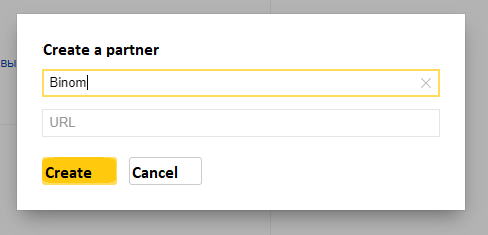In this detailed image, a user interface is displayed prominently featuring a search or text input bar. Positioned within the input bar, the incomplete word "BINOM" is being typed, indicated by the visible blinking typing cursor at the end of the text. Above this input field, a label reads "Create a Partner," guiding the user's action. Beneath the input bar, three distinct buttons are present, each labeled respectively as "URL," "Create," and "Cancel." The interface showcases a clean and vibrant color scheme, utilizing shades of black, white, yellow, green, blue, and red. These colors highlight various elements, making the interface both functional and aesthetically pleasing.